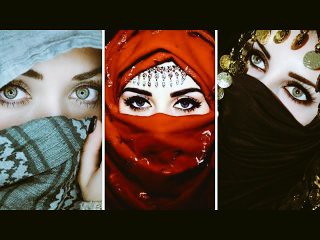This striking composite image showcases three color photographs of women whose faces are veiled, revealing only their eyes and eyebrows. Each photo is bordered at the top and bottom by a thick black line. On the left, a woman with vibrant pale blue eyes and well-trimmed dark eyebrows is seen. She wears a light blue headscarf and covers her lower face with a blue and green patterned fabric, holding it up with a hand that displays a black-painted thumbnail. The central image features a woman with intensely dark eyes, possibly black or dark brown, framed by dark eye makeup and thick penciled brows. Her head is wrapped in a red scarf that also veils her nose and mouth, with a string of jewels cascading from beneath the scarf over her forehead. The right photo presents a woman with striking green eyes, dark eyebrows, and pronounced black eyeliner and mascara. Her nose and mouth are concealed by a black scarf, and her headwear includes a collection of decorative pendants. These adornments, some gold and at least one green, hang over her forehead and trail down the left side of her face. The unifying theme across all three images is the captivating focus on the women's eyes, framed within their variously colored and decorated veils.